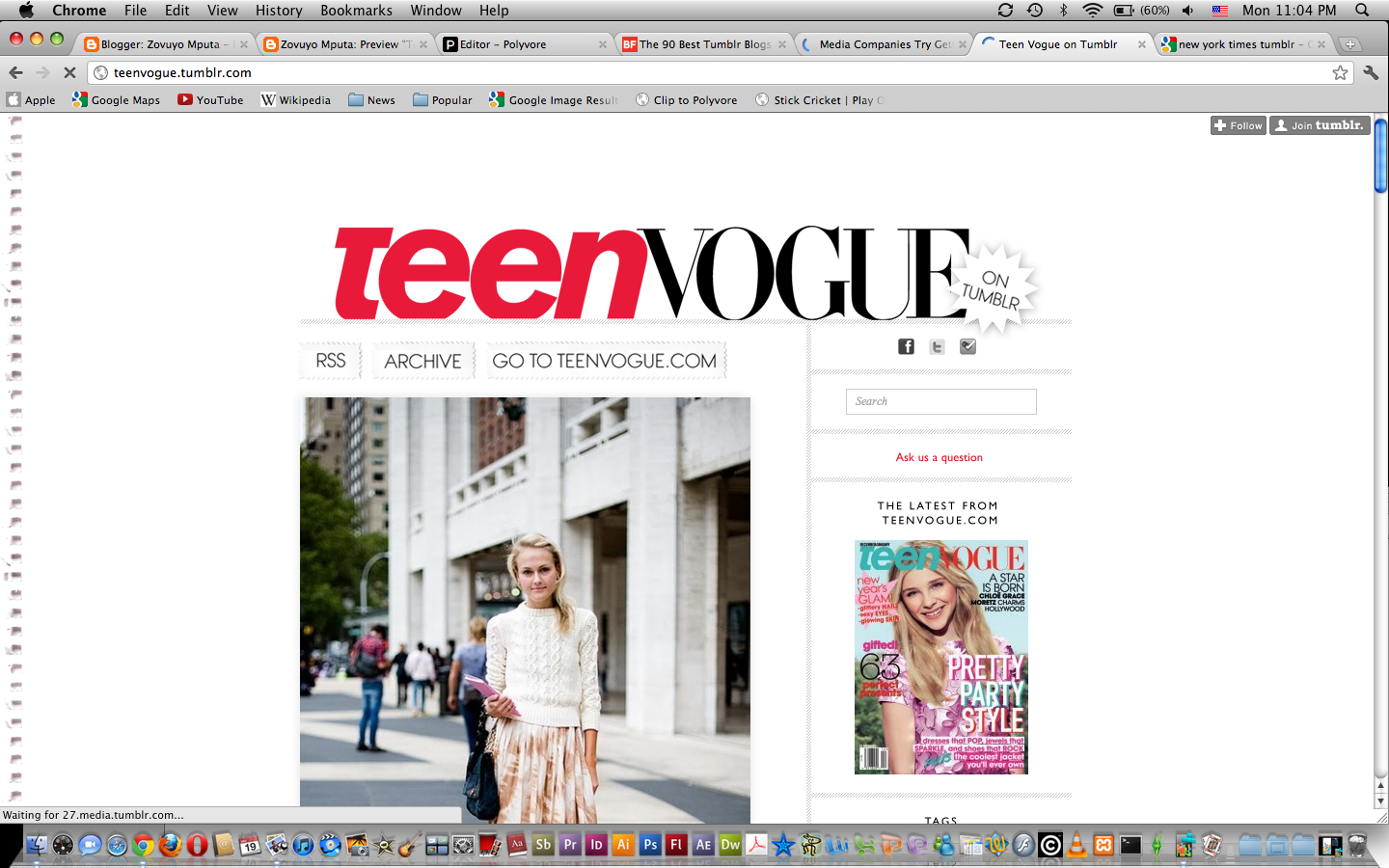This is a screenshot of an Apple Safari browser, displaying seven open tabs. The first two tabs are from Blogger, the third from Polyvore, and the fourth from BF. The fifth tab is a media company search engine, followed by the sixth tab, which is Teen Vogue on Tumblr, and the seventh tab, the New York Times Tumblr. 

The active webpage shown in the screenshot is the Teen Vogue Tumblr page, characterized by a clean, white background. At the top-center of the page, "Teen Vogue" is prominently displayed, with "Teen" in red and "Vogue" in black, giving it a unified look as a single title. 

Below the title, there is a photograph of a woman with blonde hair, dressed in a crocheted long-sleeve cream sweater and a brown-and-white patterned skirt. She is accessorized with a pink notebook and a velvet bag with a gold chain handle, suggesting a stylish yet casual outfit. The setting appears to be an urban plaza, bustling with people and surrounded by tall skyscrapers.

On the right side of the webpage, there is an image of the latest cover of Teen Vogue featuring actress Chloe Grace Moretz. The cover headline reads "Pretty Party Style" and highlights sections such as "63 Perfect Presents" and "A Star is Born: Chloe Grace Moretz Charms Hollywood."

At the bottom of the screenshot are various icons, which are part of the computer's interface rather than the webpage.

This detailed caption provides a clear and thorough description of the screenshot, its contents, and the context within the Safari browser's layout.